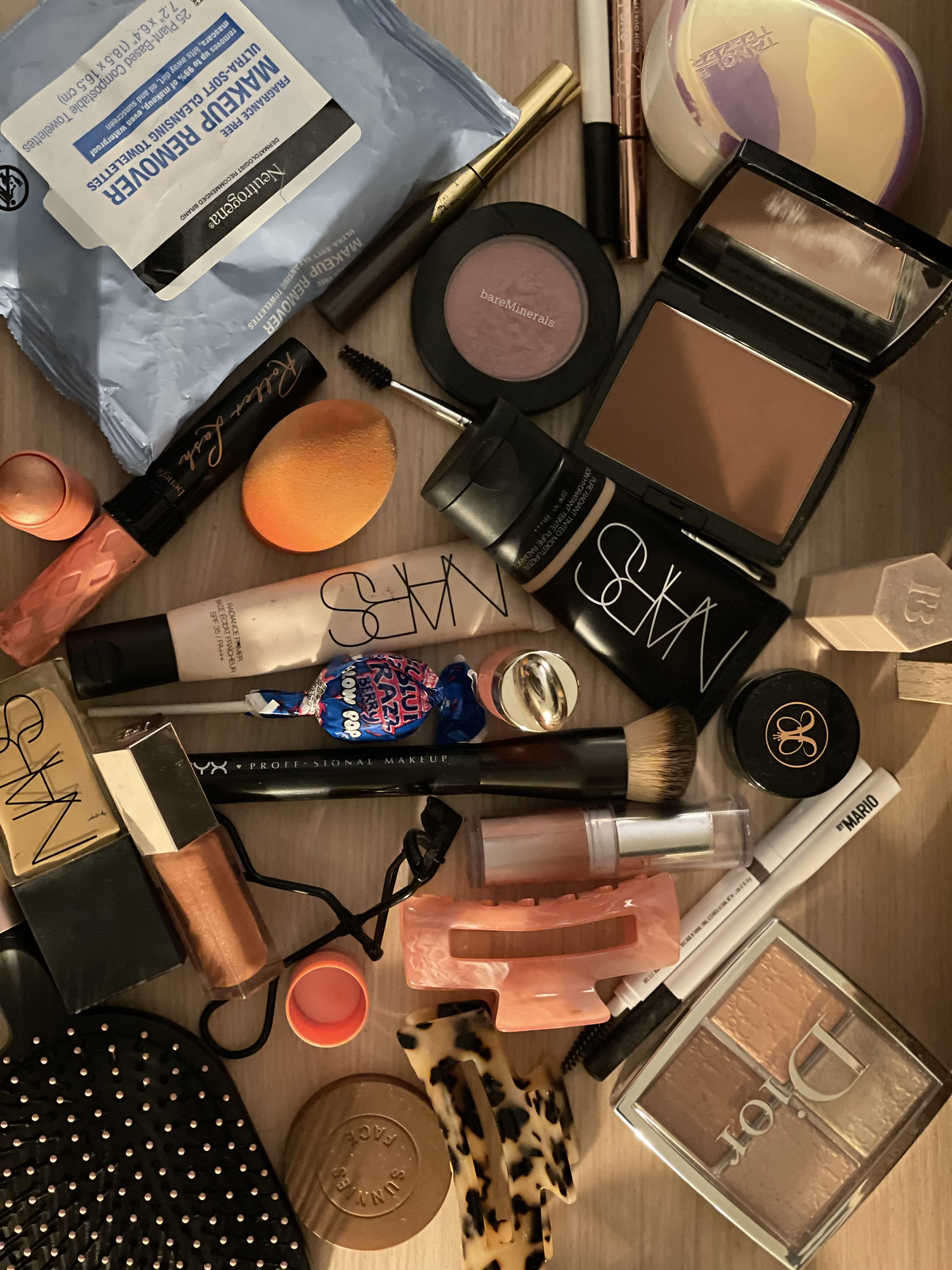On a nearly white, light brown wooden table, various items appear to have been hastily dumped out from a purse. Dominating the scene are numerous cosmetics alongside a few other personal items. A paper-wrapped Blow Pop lollipop, a pink hair clip, a ballpoint pen, and a fine point marker pen are scattered among the cosmetics. A scissor-shaped eyelash curler lies amid the clutter, a relic from childhood recognition. A flexible pack of Neutrogena makeup remover towelettes provides a practical touch.

Among the cosmetics, an array of products can be seen. A Bare Minerals compact, featuring a brown rim, black lip, and clear top with the logo printed on it, reveals a pink cosmetic disc inside. An open rectangular case with a mirror in the lid and dark tan makeup inside stands out. Two tubes of NARS cosmetics, one cream-colored with black text and writing too small to read, the other black with white text and a tan band, add a touch of sophistication. Another NARS item, a black square case with a clear top and a tan-looking product inside, is also visible. 

A makeup brush sporting the brand "NYX Professional Makeup" adds to the mix, while a Dior cosmetic set, encased in a square case with a silver rim and clear lid, showcases four shades ranging from cream to brown. Additionally, an oval makeup sponge and a bottle of nail polish round out the assortment. This chaotic yet revealing collection tells a story of everyday beauty routines on a textured wooden stage.